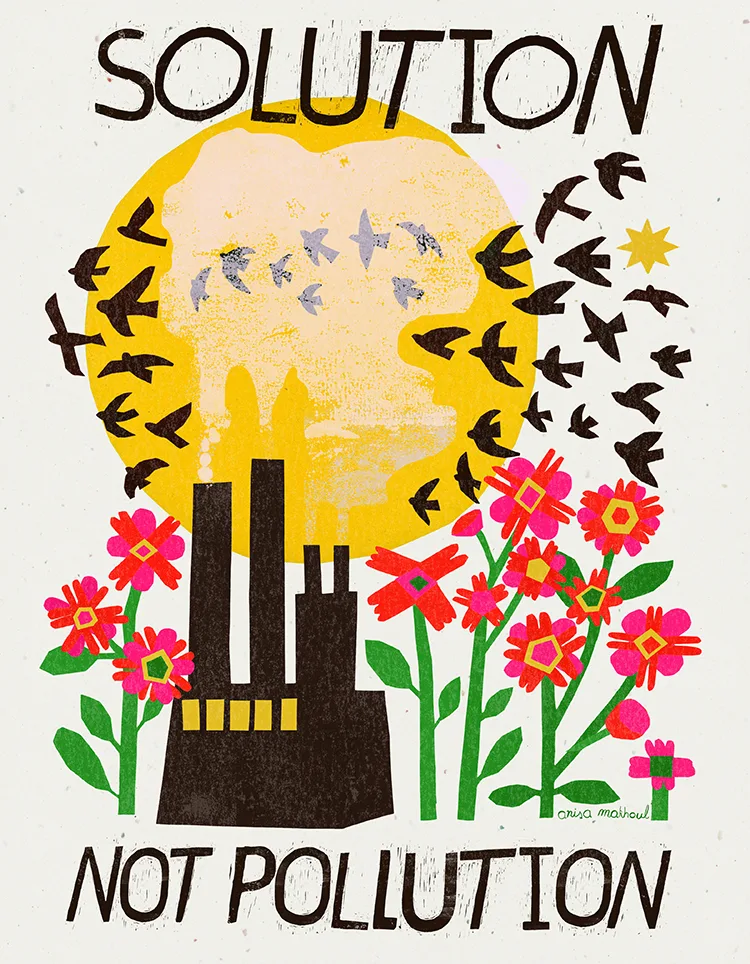The image is a promotional poster designed without a border and featuring a vertically rectangular layout with a predominantly off-white or light gray background. At the very top in bold, black, all-capital letters, it reads "SOLUTION," and at the very bottom, similarly stamped, it says "NOT POLLUTION." 

Central to the poster's design is a large, illustrated yellow sun dominating the upper portion, with approximately two dozen black, blocky birds flying across it. To the left of the sun appears a smaller, yellow star in the corner. Beneath this sun, a factory stands in silhouette with four large smokestacks emitting thick, white smoke that extends upward, partially obscuring the birds and blending into the sky. On both sides of the factory are green-stemmed flowers with pink and orange petals and yellow centers, adding a contrasting natural element to the industrial scene.

Overall, the image employs vivid colors and high-contrast elements to deliver a clear and impactful message promoting environmental awareness.